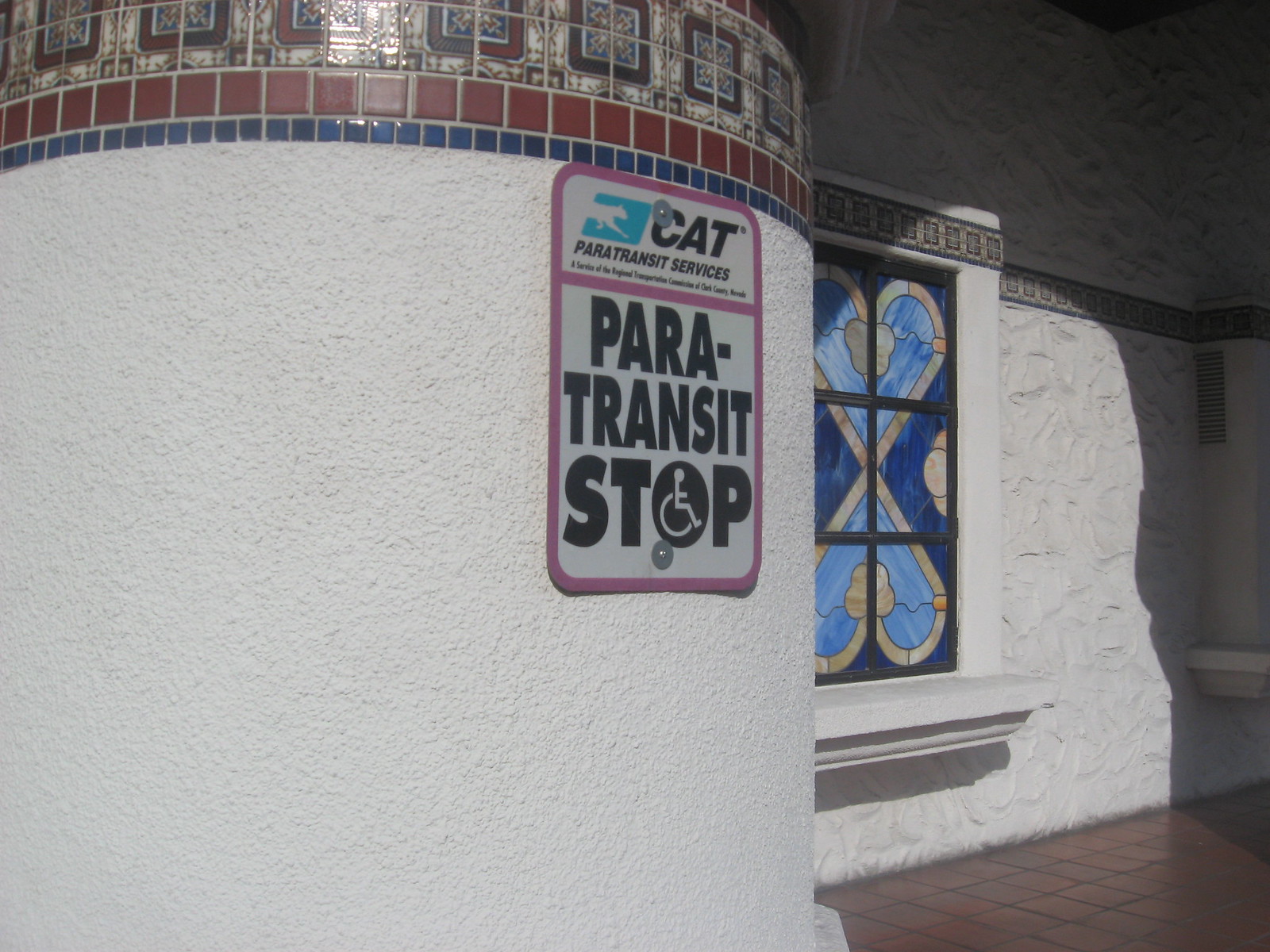This outdoor image captures a side view of a stucco building taken from an angle. The structure prominently features a cylindrical section and a rectangular section, both coated in white stucco with distinct textures. The cylindrical part boasts a popcorn texture, while the rectangular part has a more traditional rough texture. Atop the cylindrical section, there is an intricate geometric design made up of cream and maroon-colored tiles with splotches of blue. These tiles form a series of different sized squares in a layered pattern, culminating in smaller maroon and blue tiles beneath.

Central to the image is a rounded rectangular sign with a pink border and white background, displaying "Paratransit Stop." Notably, the "O" in "Stop" contains an icon of a disabled person in a wheelchair. Above this, there is another sign that reads "Cat Paratransit Services," accompanied by a blue and white icon. The sign appears to be affixed to the cylindrical part of the building.

To the right, a stained glass window featuring various shades of blue in symmetrical vertical heart patterns is visible. The presence of sunlight casts shadows on the wall, adding depth to the scene. Additional elements in the background include a vent and floor tiles that appear to be either red or orange.